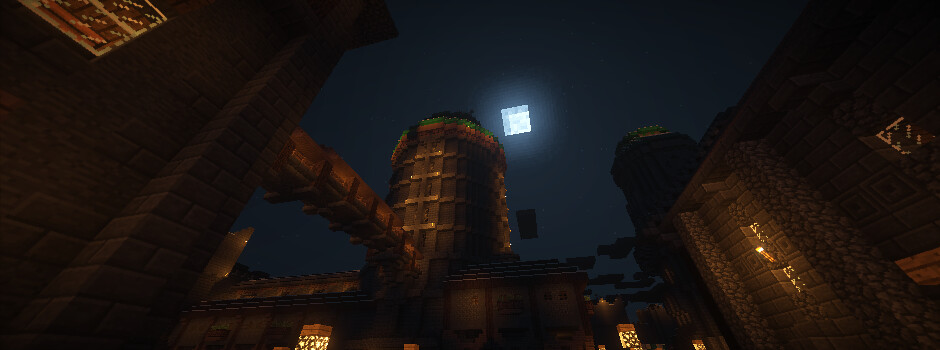This captivating nighttime screenshot from the computer game Minecraft showcases a stunningly detailed scene. The view is from the ground looking up towards the sky, which is a deep, dark blue. The area appears to be castle-esque, with brown and orange-hued buildings, giving off a warm, illuminated glow from their windows. Dominating the scene are two prominent brown pillars or towers, connected by a bridge, creating a majestic architectural silhouette against the darkened sky. To the left, a rectangular window in a tower emits a soft orange light. The most striking feature is the bright white, square-shaped moon that brilliantly lights up part of the sky, adding to the night-time ambiance of the scene. Various structures with their tower-like forms and rugged, blocky texture emphasize the game’s distinct cuboid aesthetic, enhancing the image's immersive and enchanting atmosphere.